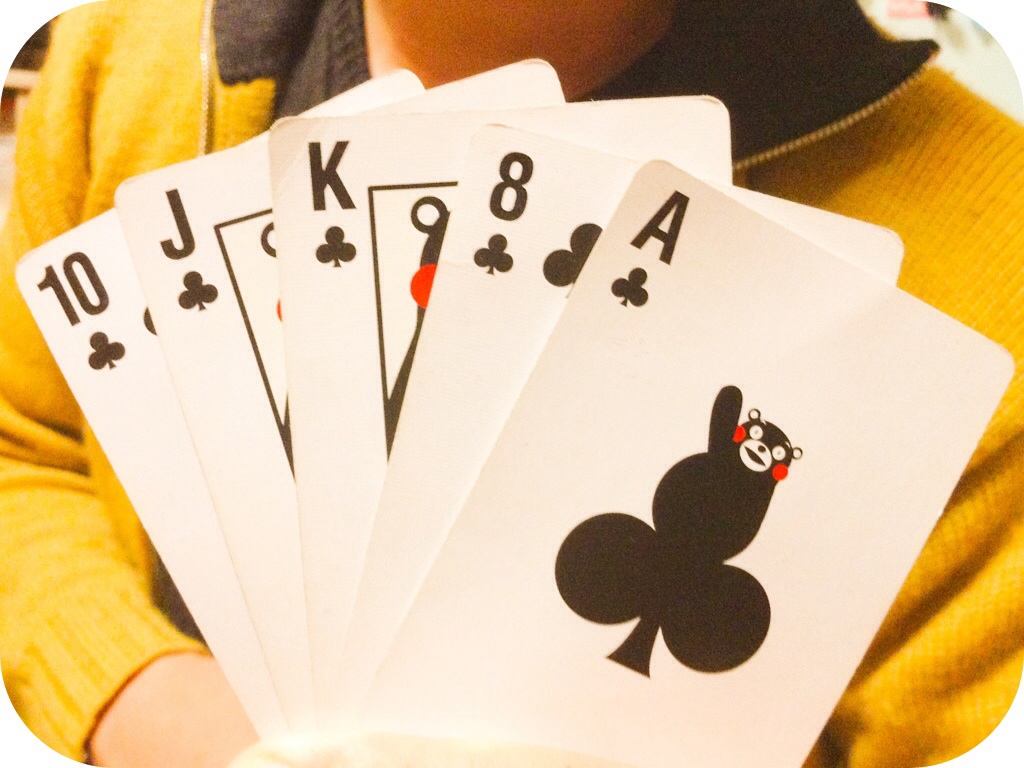The image is a close-up shot featuring the lower part of a person's neck, their shoulders, and chest. The individual is wearing a yellow sweater with a black interior around the neck, layered over a black shirt. The sweater appears to have a zipper at the top. The person is holding five playing cards in front of them, with their hands partially visible. 

The cards, all from the suit of clubs, are arranged in a fan-like spread. The visible cards are the Ace, Eight, King, Jack, and Ten, with the Ten positioned at the back of the pile. Uniquely, the King card does not depict the usual royal image but instead features a cartoon bear. The bear is illustrated with red circles for cheeks, eyes, a nose, a mouth, and little ears. One of the bear’s arms is raised, as if waving. The character’s body is integrated into the club symbol, with the top part of the club resembling the bear’s circular body.